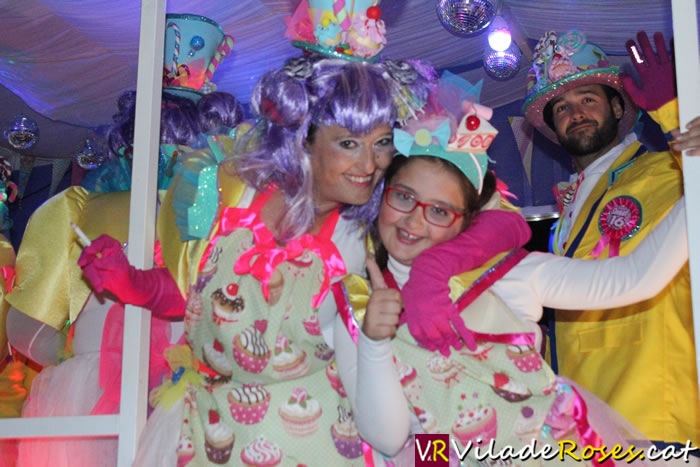In the vibrant and whimsical photograph, a group of people are dressed in quirky, colorful costumes that evoke a playful, candy-themed atmosphere. Central to the image is an older woman, likely in her 40s, wearing a shiny purple wig, a dress adorned with cupcake prints, and long pink gloves. She has her arm affectionately wrapped around a smiling young girl, approximately 10 years old, who sports a playful paper hat decorated with cake and candies, giving a cheerful thumbs up. Both are beaming at the camera, creating a warm and joyful focal point. 

The younger girl wears red glasses and a matching dress with cupcake designs, complemented by a cream long sleeve shirt. To the right stands a man in a striking yellow suit coat, topped with a festive lollipop hat, and a bright pink ribbon pinned to his chest. His exuberant outfit harmonizes with the overall lively theme of the scene. In the background, other individuals in similarly extravagant and candy-themed costumes, complete with elaborate hats featuring candy designs, add to the festive atmosphere. The image is captioned in the bottom right corner with the text "VRVilladeRoses.cat," highlighting the jovial nature of this candy-coated celebration.